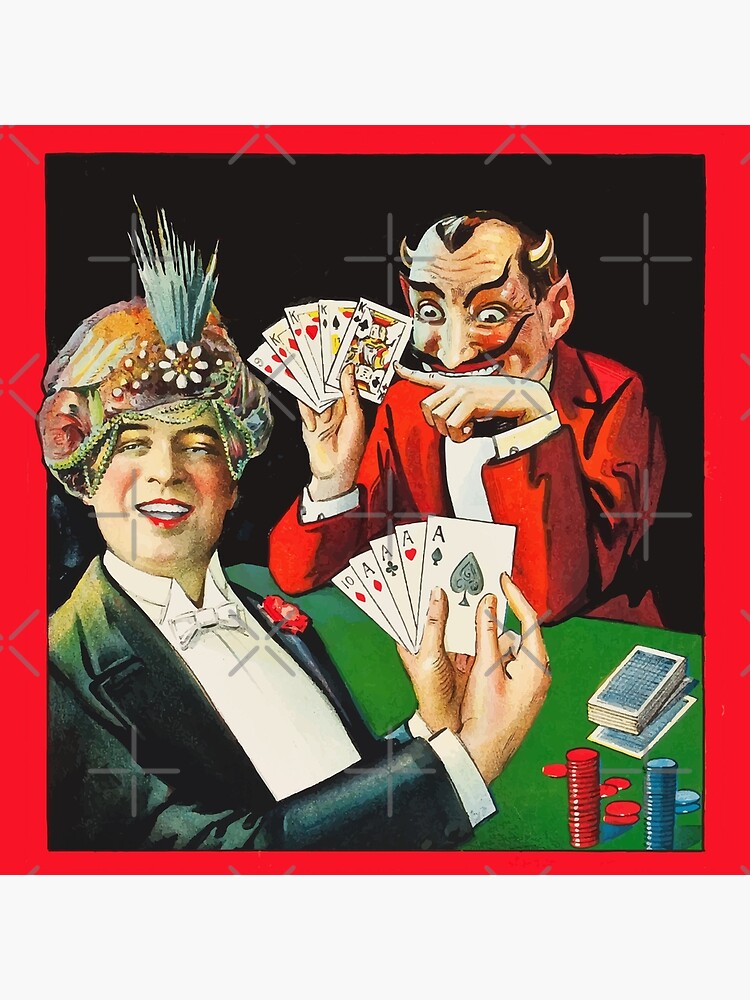In this detailed cartoon image, we see two central figures engaged in what appears to be a lively game of poker at a green table. On the left, there's a person with a large, ornamentally decorated headdress featuring flowers, beads, and fruits. This individual, wearing a black jacket and red lipstick, is prominently displaying their hand of four aces and a ten towards the viewer, with a red rose pinned to their suit pocket. 

To the right, there is an imposing figure dressed as the devil, characterized by his red blazer, white dress shirt, black mustache, horns, and pointed ears. This devilish character is delightedly pointing to his own hand of four kings and an eight of hearts, smiling broadly with large eyes. The background is stark black, outlined in red, enhancing the dramatic atmosphere. Below the deck of cards on the table, neatly stacked, are red and blue poker chips, adding more color to the scene. This imaginative and detailed illustration, reminiscent of something out of a New Yorker magazine, captures a whimsical yet intense moment in the game.